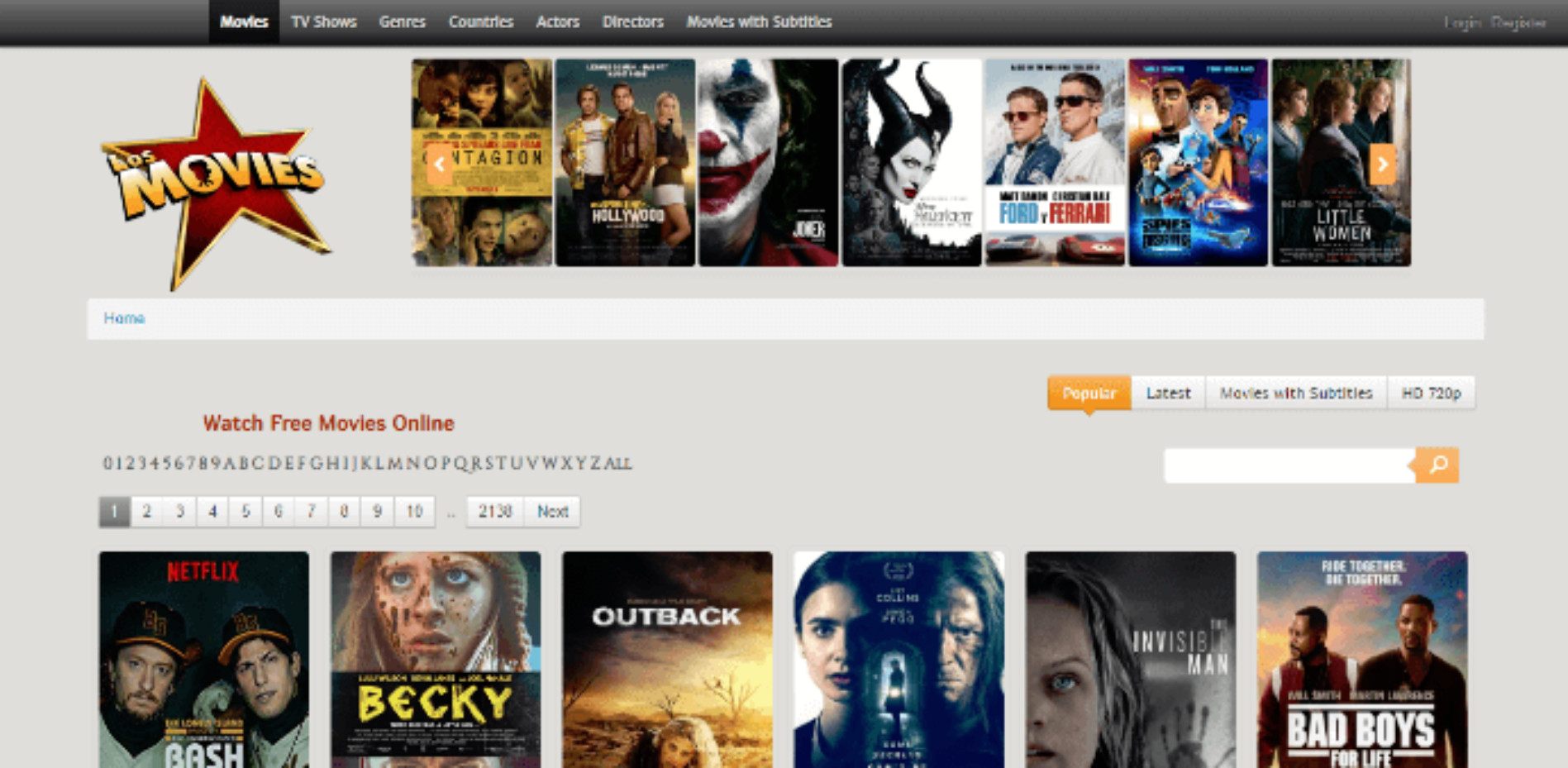The image is a screenshot from a movie streaming website, showcasing its interface. At the very top, the site features a navigation menu set against a dark gray background. The menu items are written in white, listing "Movies Now" (highlighted in black as the current page), "TV Shows," "Genres," "Countries," "Actors," "Directors," and "Movies with Subtitles." These options provide various ways to browse the content library.

The website's background is a light gray hue. Prominently displayed at the top is the website's logo, which includes a red star outlined in gold next to the word "MOVIES" in all capital letters written in a gold font. The letter "O" in "MOVIES" is creatively replaced by a tiny illustration of an old-style movie projector.

Below the navigation menu, the site showcases movie posters in a row. The first row includes several films like "Joker," identifiable by the haunting image of the Joker’s white-painted face, and "Ford v Ferrari." Beneath this row, a second row displays additional movie titles, including "Bad Boys for Life" in the lower right corner and "Outback" in the center.

Between these rows, two columns of text are displayed in red font. On the left, it says "Watch Free Movies Online." On the right, another menu features categories for sorting content: "Popular," "Latest," "Movies with Subtitles," and "HD 720p" quality options.